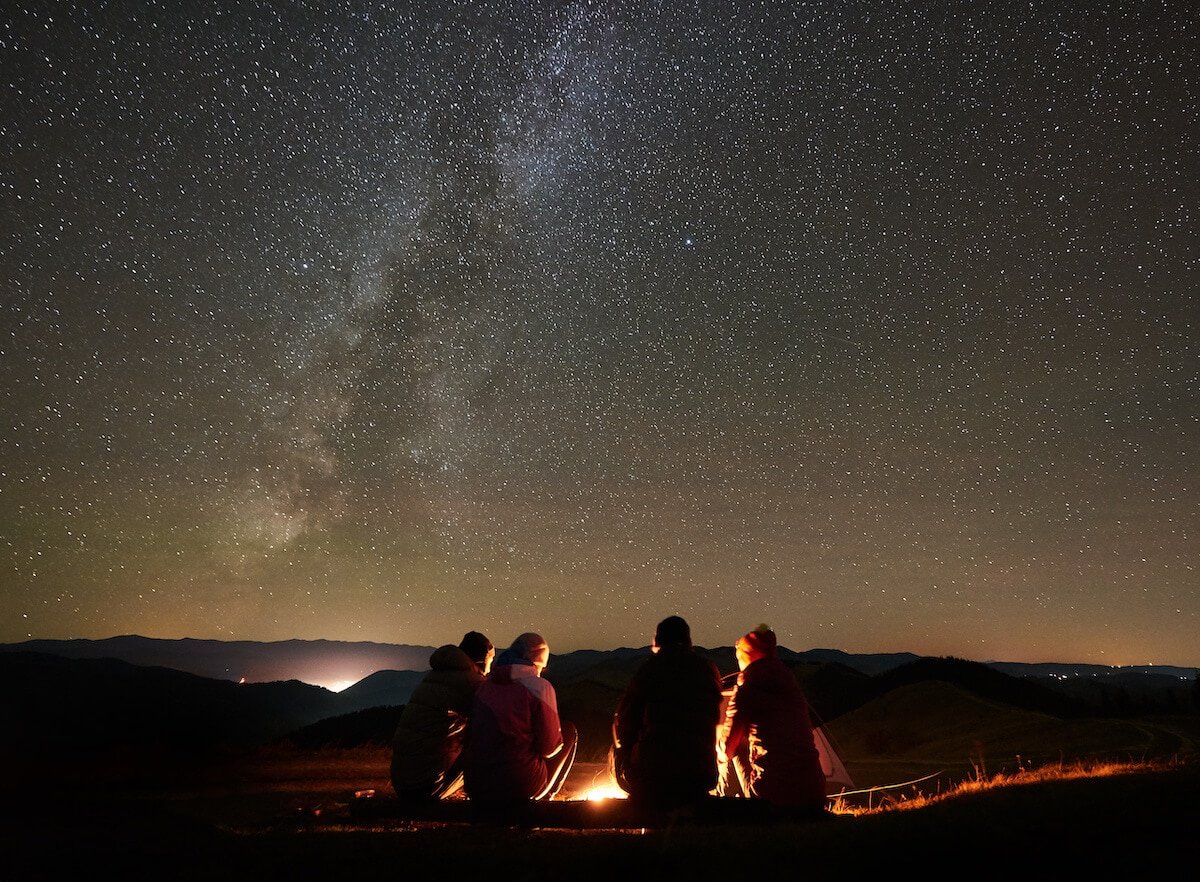A detailed photo captures an outdoor night scene where four people, appearing to be two couples, are seated on a long tree trunk in a grassy area. They are illuminated by the warm glow of a bonfire, with the light revealing one person in a dark coat and another in a reddish jacket, all dressed warmly for the cold. Behind them stretches a breathtaking night sky, filled with grayish hues and countless white spots resembling stars. The sky casts a serene backdrop, dotted with silhouettes of distant mountains. A light can be seen far in the valley between the mountains, possibly hinting at a far-off city. The overall ambiance suggests a peaceful camping outing under a star-studded sky.